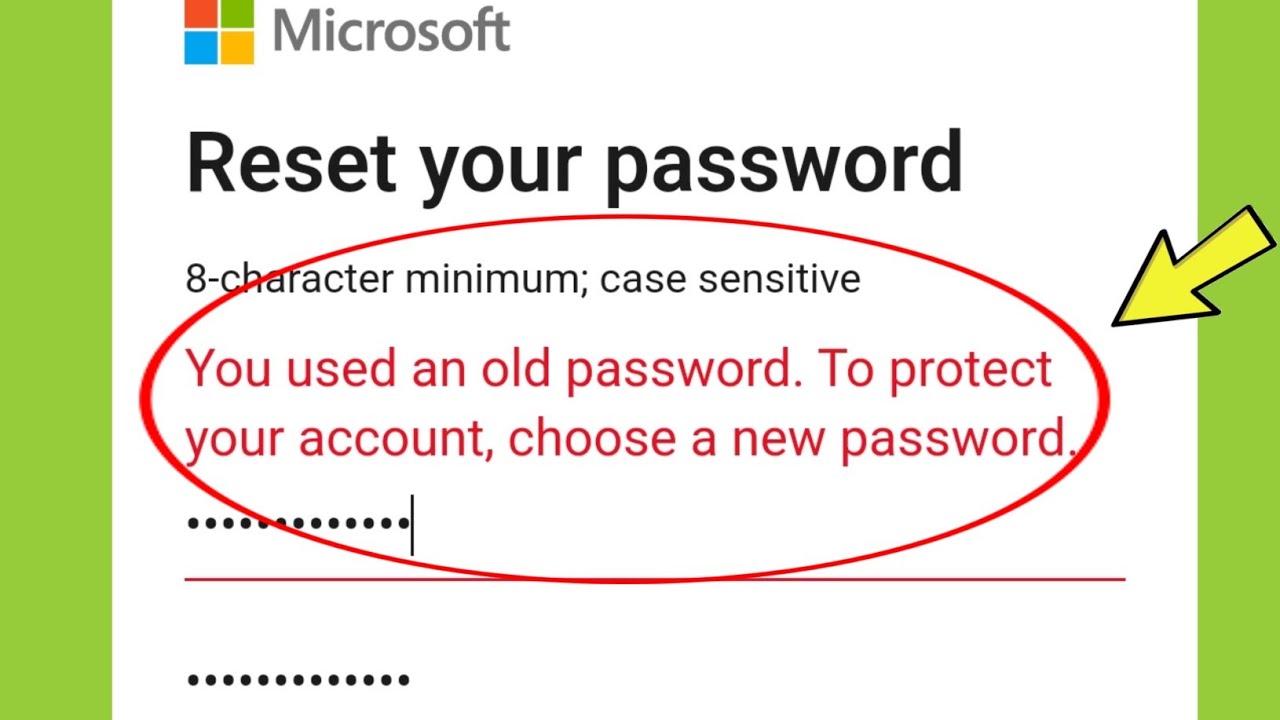The image appears to be a screen capture, likely taken from a cell phone or a smaller section of a webpage on any size monitor. The screen grab is characterized by a lime green bar on both the left and right sides, framing a central white box. 

At the top left corner of the white box, the iconic Microsoft logo is prominently displayed, featuring its four-color panel with red and green on the top, and blue and yellow on the bottom. Positioned to the right of the logo, "Microsoft" is written in gray text. Immediately below the logo, bold black text reads "Reset Your Password," followed by instructions in smaller black text that states, "8-character minimum, case sensitive."

A significant section of this white background area is highlighted with a red circle, emphasizing an error message in red text: "You used an old password to protect your account, choose a new password." A visual confirmation that the user has attempted to enter their password twice is provided by two rows of black asterisks just beneath the error message.

On the right center of the image, a large black-outlined yellow arrow extends from the lime green background bar, directly pointing towards the red error message, drawing attention to the need for the user to choose a new password.